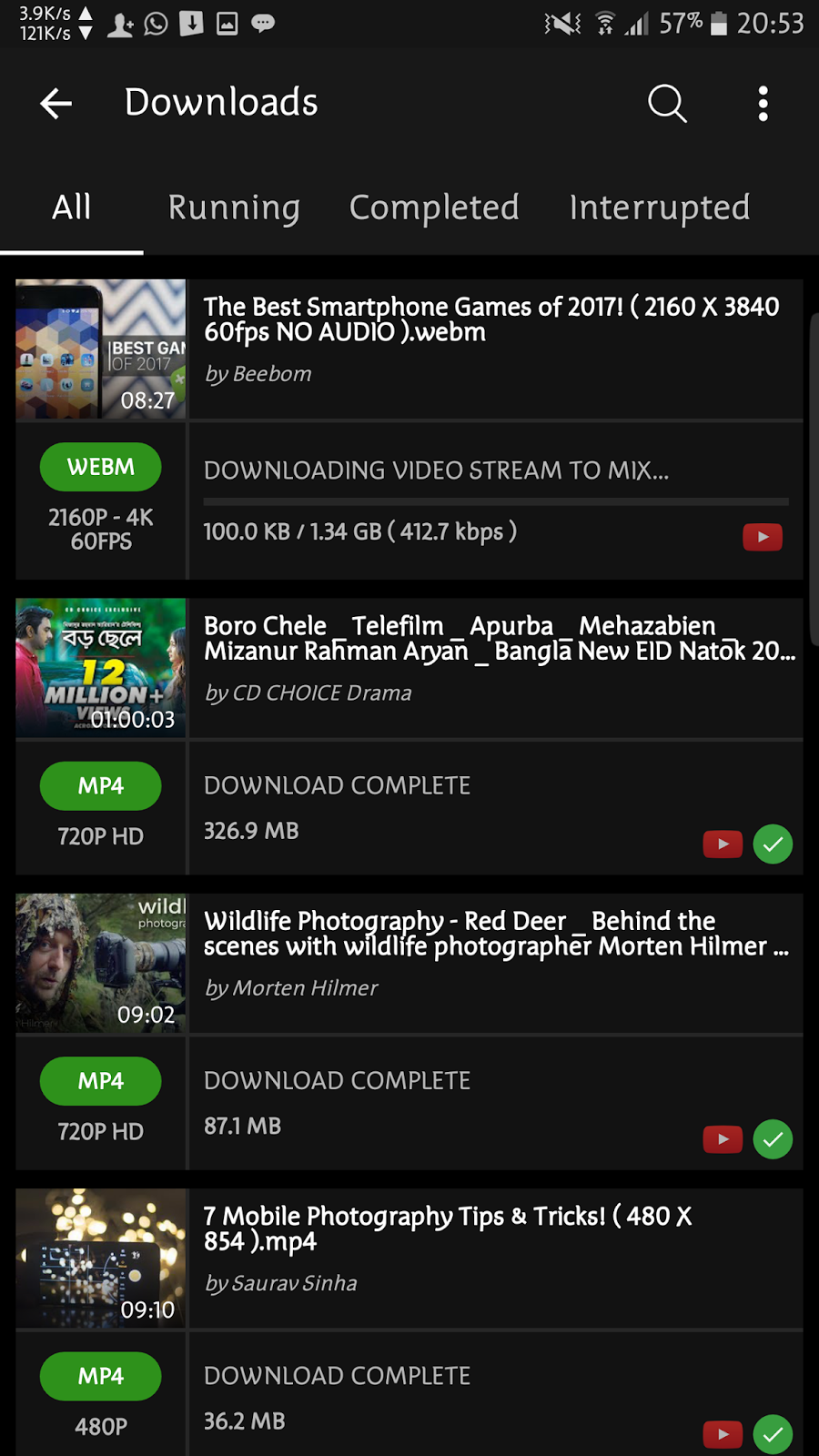This mobile screenshot captures a moment at 20:53, as indicated at the top right corner. The battery life at the time is 57%. Various icons are visible on the right side of the status bar, showing signal strength, battery life, and other statuses. On the left side, there are indicators for ongoing downloads and background apps.

The screen has a dark gray background with white and light gray text. At the top, the header reads "Downloads," accompanied by a back arrow button on the left. To the right of the header, there are icons for a magnifying glass and a vertical three-dot menu, which typically denotes additional options or settings. 

Below the header, different tabs like "All," "Running," "Completed," and "Interrupted" categorize the downloads. 

The main section of the screen displays a list of various files being downloaded, including three MP4 videos. The titles of the files suggest they are saved from YouTube, with names like "The Best Smartphone Games of 2017."